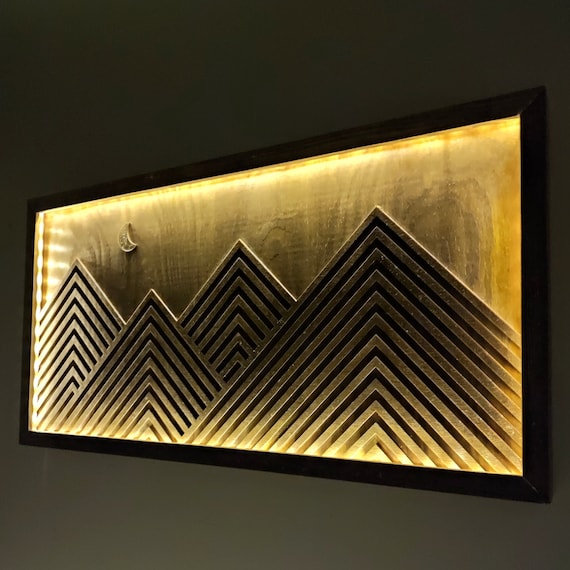In this image, an intricate sculpture hangs on a dimly lit, gray-colored wall, evoking an air of sophistication. The rectangular artwork is framed in a dark, possibly black or wooden frame, adding to its elegance. Inside the frame, the sculpture features four meticulously carved, triangular pyramids resembling mountain peaks, arranged in distinct lines. These pyramids, along with a crescent moon above them, are crafted from a dark, golden-hued metal, giving the piece a luxurious, sand-dune-like appearance. The sculptures are brightly illuminated by internal yellow lights, highlighting the carvings and golden background. The overall impression is one of opulence, suggestive of a decoration that would befit a wealthy individual's home or business.